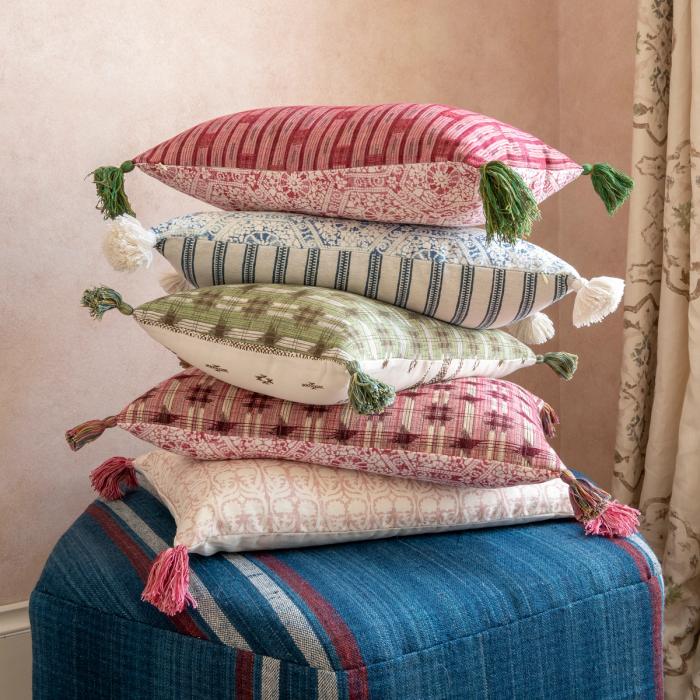In the image, there is a stack of five rectangular pillows, each adorned with tassels at the corners. The pillow at the bottom features tassels in a pinkish hue. The second pillow from the bottom has multicolored tassels consisting of pink, blue, and green shades. Moving upward, the third pillow's tassels are green, followed by the fourth pillow with white tassels. The top pillow in the stack again has green tassels. 

On the right side of the image, partially cut off, are curtains made of a fabric that appears to be a mix of beige and olive green. The wall behind the pillows is beige, and a white baseboard is visible at the lower left-hand side of the image. The pillows are resting on a soft surface, likely an ottoman, that is predominantly blue with red and white stripes, although the image is zoomed in closely, limiting the view.